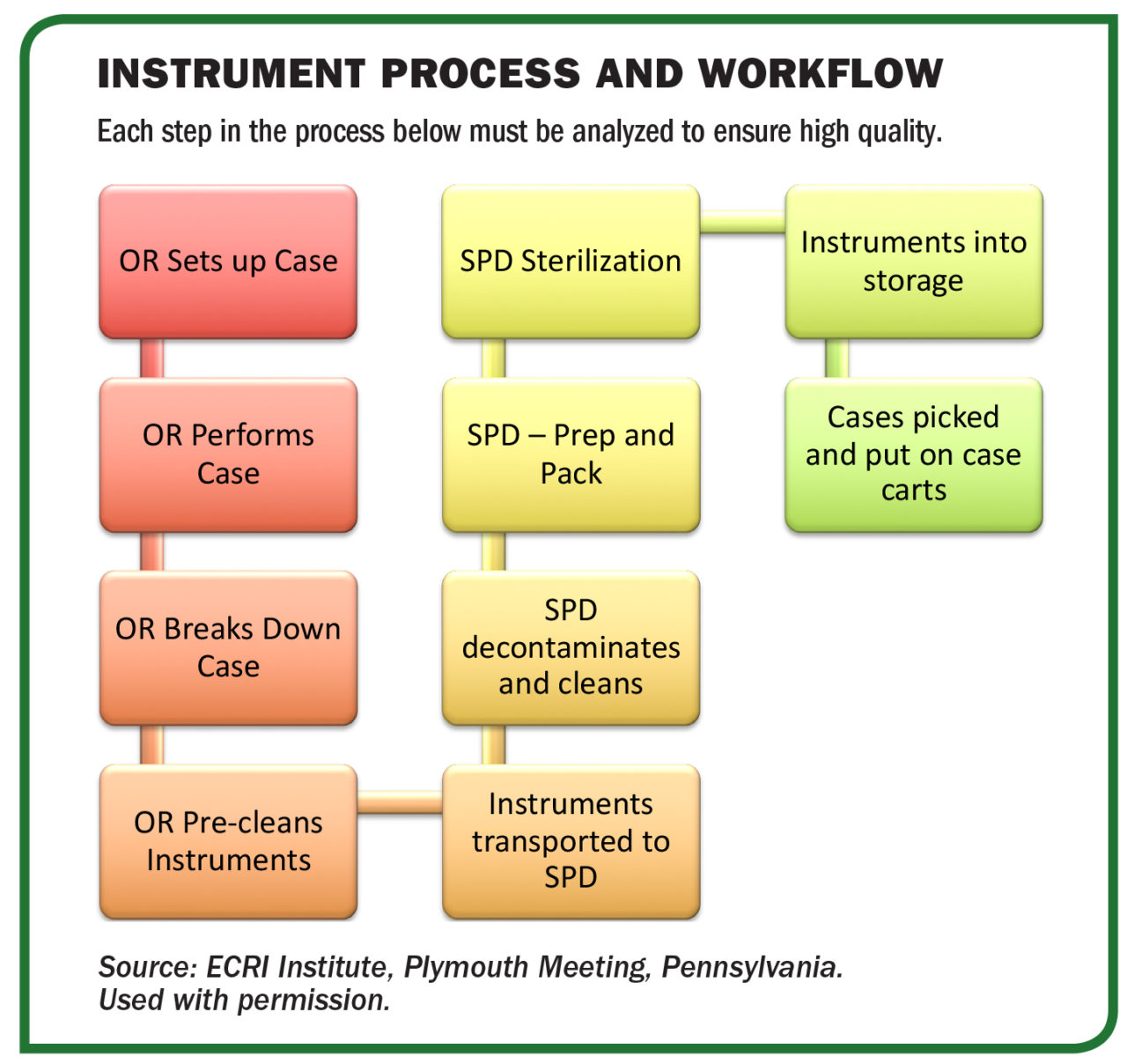This detailed poster titled "Instrument Process and Workflow" features a flowchart describing the sequential steps involved in a particular process, potentially the sterilization of medical instruments. Bold black letters at the top state the title, and a subtitled note emphasizes that "Each step in the process below must be analyzed to ensure high quality." The flowchart moves left to right, and vertically up and down through various stages, starting with steps such as "OR sets up case," "OR performs case," and "OR breaks down case." The background color of the boxes transitions from red to orange, then yellow, and finally lime green, indicating a progression or categorization of steps. At the bottom, the chart cites its source: "ECRI Institute, Plymouth Meeting, Pennsylvania," noting that the information is "used with permission." This educational tool is likely used in classrooms or textbooks to instruct on the detailed workflow and high-quality analysis required in the instrument process.